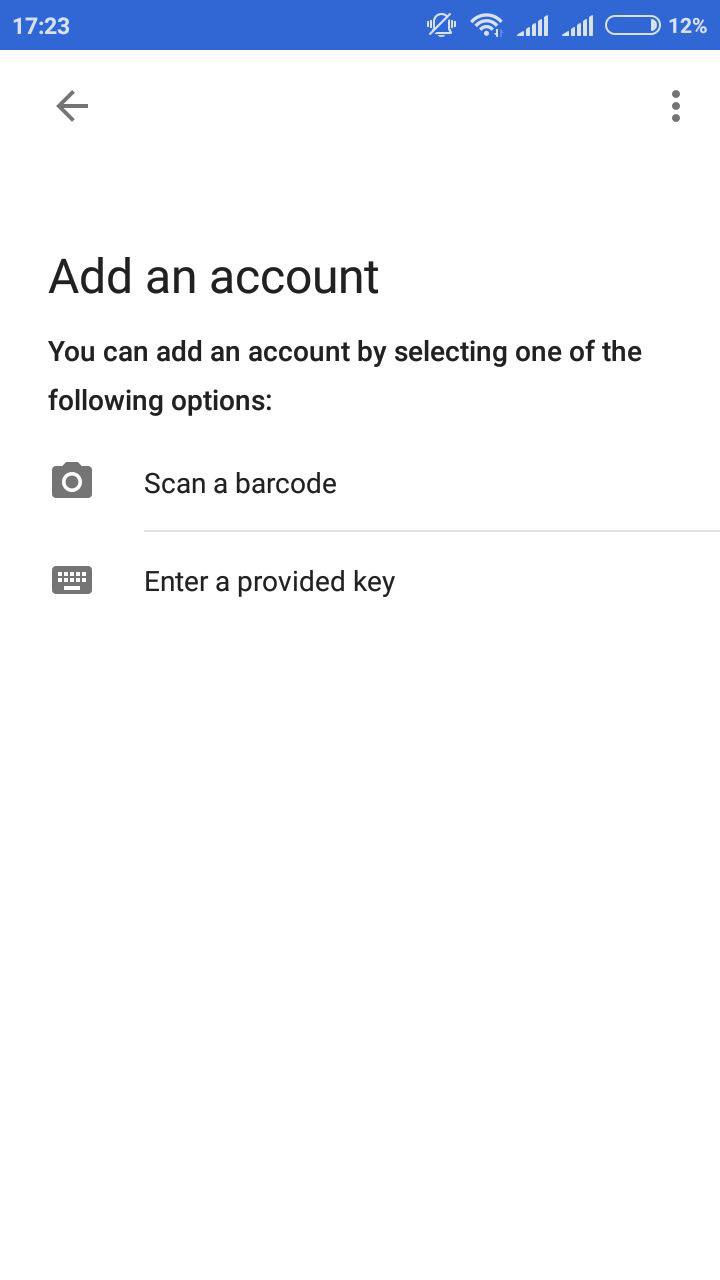The image captures a screenshot taken from a cell phone. At the very top of the screen, there is a light blue rectangular line displaying the time as 17:23. Moving to the right, various status icons are visible, including a Wi-Fi symbol, a crossed-out notifications icon, two triangular bars indicating signal strength, and a battery icon with 12% remaining, shown with a small amount of white in a blue battery indicator.

Beneath the status bar, there is a gray arrow pointing to the left, followed by three vertical gray dots representative of a menu or options button. Further down, the screen displays the text "Add an account." Below this, there is a prompt stating, "You can add an account by selecting one of the following options."

Two illustrated methods are provided for adding an account: 
1. A gray camera icon with the text "Scan a barcode."
2. A keyboard icon with the text "Enter a provided key."